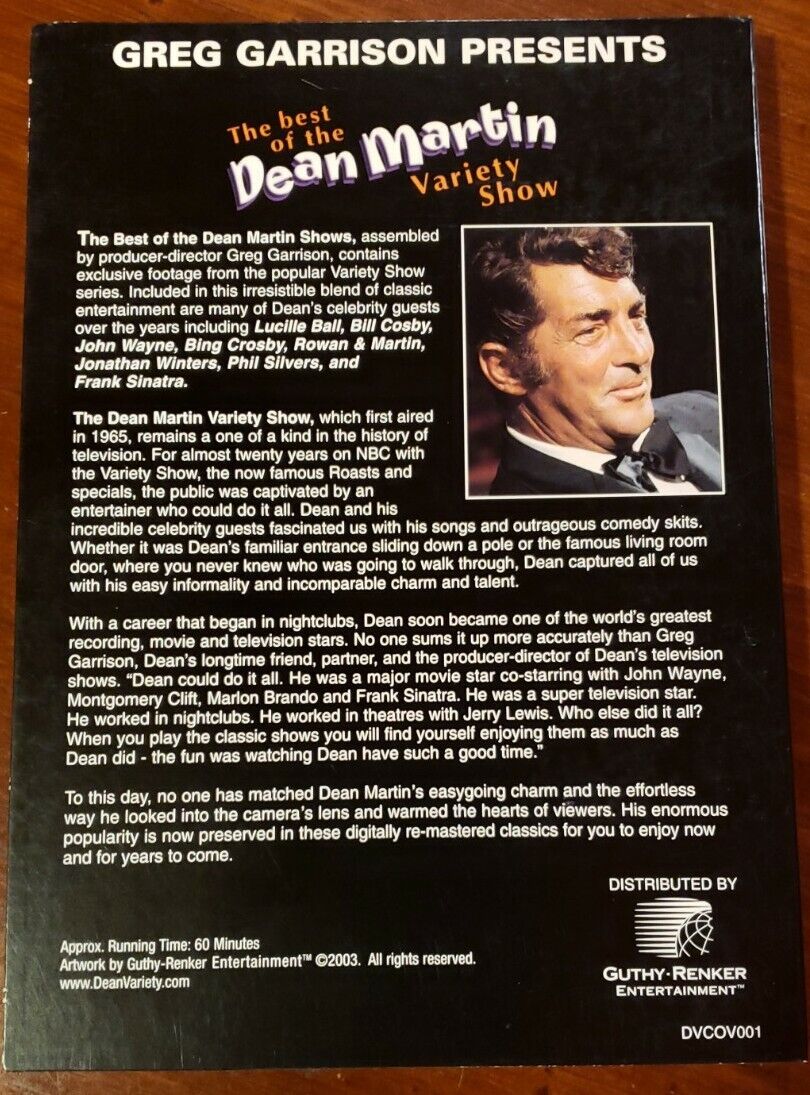This advertisement, resembling the back cover of a VHS tape, features a vertical, rectangular design with a dominant black background. At the top, in bold, uppercase white letters, it reads "Greg Garrison Presents." Just below that, in a stylish, irregular handwritten font, "Dean Martin" is prominently displayed, with "the best of the Dean Martin variety show" in smaller orange letters.

A color photograph of Dean Martin in a tuxedo is positioned on the upper right-hand side, capturing him looking distinguished and to the right. This photo injects vibrancy into the layout, standing out against the black backdrop.

Beneath the headline and photograph are four paragraphs of much smaller white text, meticulously detailing the renowned Dean Martin variety show, along with descriptions of the various actors featured.

At the very bottom of the frame, essential details such as the running time and artwork credits are provided, marked with the copyright 2003. In the lower right-hand corner, the logo of Guthrie Renker Entertainment is displayed, indicating their role as the distributor.